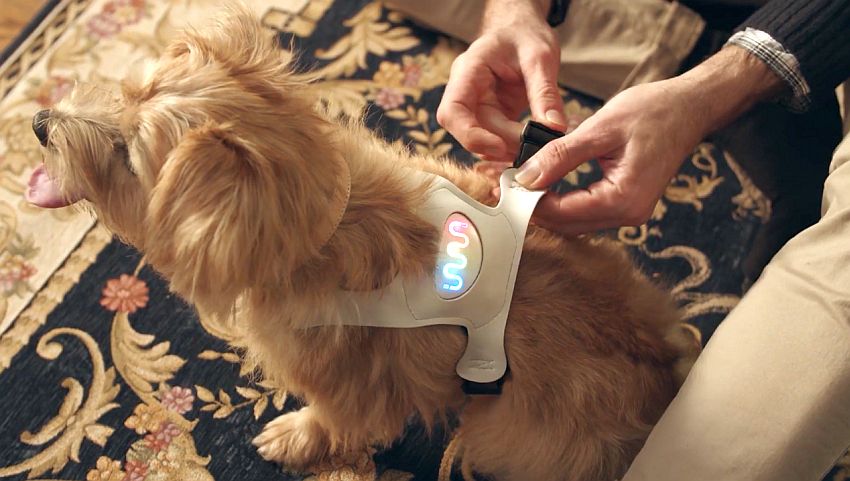This professional photograph captures a moment from above where a man is fitting a cream-colored harness onto a light brown, medium-haired terrier. The small dog, which resembles a terrier breed, stands on an ornate carpet that features a black and gold floral design, with hints of dark blue and other colors. The man’s hands, presumably elderly, are visible as he attaches the harness to the dog. The harness includes black buckles and a prominent LED display on the back, showing rainbow colors of blue, yellow, and red, designed to indicate the dog's mood. The dog stands facing left, its black nose and protruding tongue visible through the hair that obscures its eyes. Matching the dog’s fur, the harness is a cream or khaki color. The man's attire, comprising tan pants and a black sweater over a shirt, subtly complements the scene.